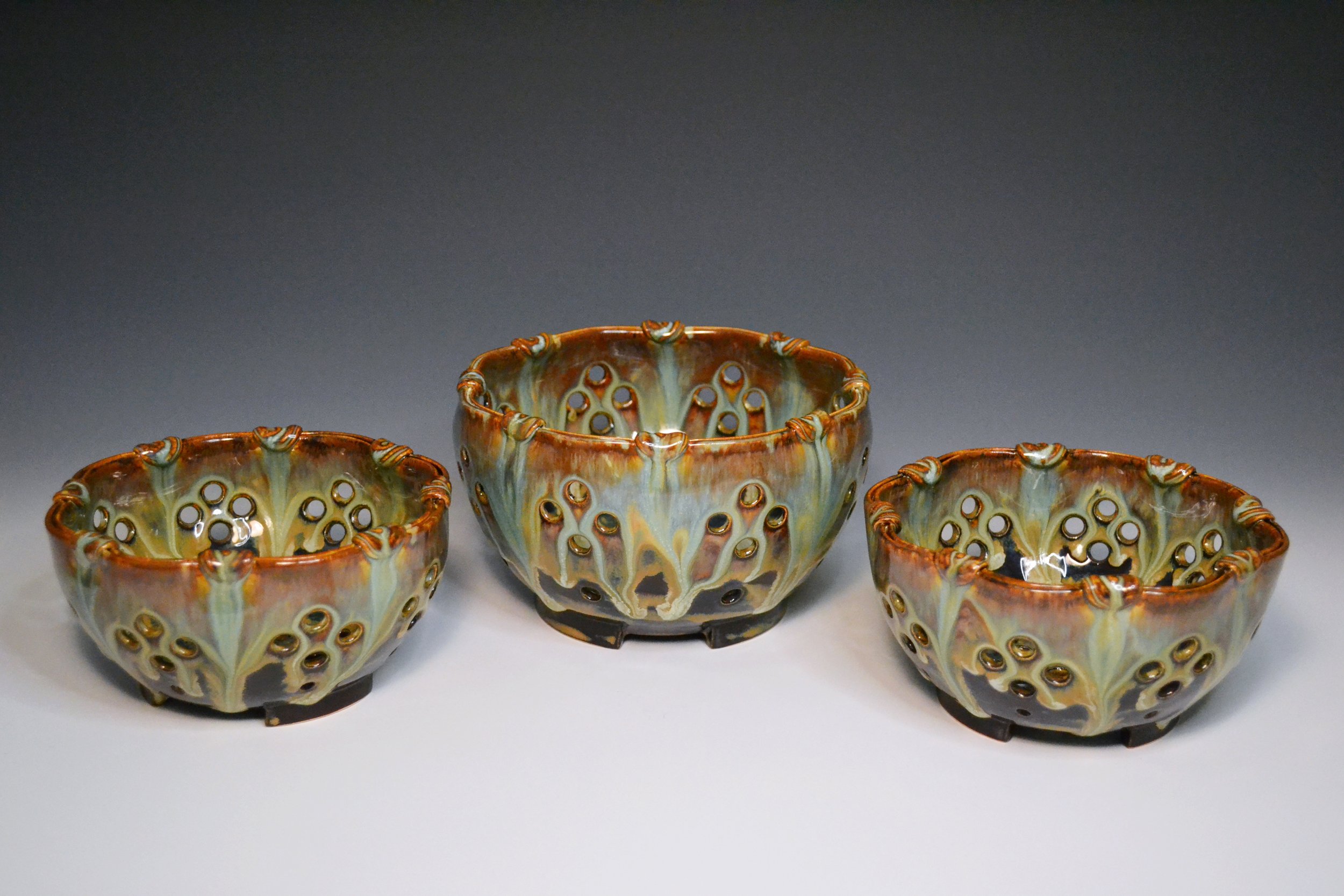This image showcases a set of three highly decorative, hand-thrown ceramic bowls, designed more for display or utility purposes than for food. The bowls exhibit a meticulously applied glaze that transitions from a rich brown at the rim to a creamy, milky white towards the base, with hints of bluish and darker tones near the bottom. Each bowl features a series of fine details, including geometric contours with eight flattened sides and several arrays of punched holes forming plus-sign shapes. These holes are evenly spaced, with one at the top, one at the bottom, and two on the sides of each panel section. One bowl is slightly larger than the other two, which match in size, creating a cohesive set. These striking bowls, set against a gray background, evoke a sense of modern artistry and are well-suited for holding trinkets or other small items.